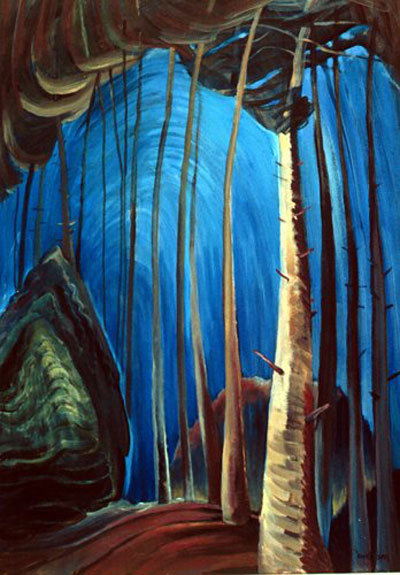This tall, rectangular painting depicts the woods at night in an abstract style. The background is a swirling, bright blue sky with hints of white, creating a circular, dramatic effect. Roughly 15 to 18 tree trunks, depicted in white and varying shades of brown, extend vertically in a non-straight manner. The dense canopy of leaves forms a dark, intricate pattern at the top of the artwork. On the left side, a large, detailed green shrub reaches midway up the painting. The ground is painted in deep red and dark brown hues, adding to the gloomy atmosphere. Additionally, there is a distinct, ornate, arrowhead-shaped stone in black and gray on the left side, enriching the textured landscape. The scene is devoid of sunlight, moonlight, clouds, animals, or people, enhancing its somber and mysterious tone.